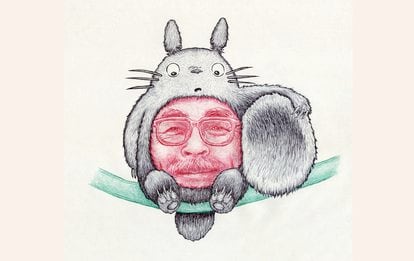The illustration depicts Totoro, a character portrayed in a minimalistic, colored pencil or ink style. Totoro is miniaturized and positioned sitting on a green strand or vine against a white background. His belly is intriguingly open, revealing the face of his creator, Hayao Miyazaki, drawn in red with glasses, a mustache, and a smile. Totoro appears concerned, gazing down at Miyazaki's peeking face from his belly, creating a whimsical and curious scene.